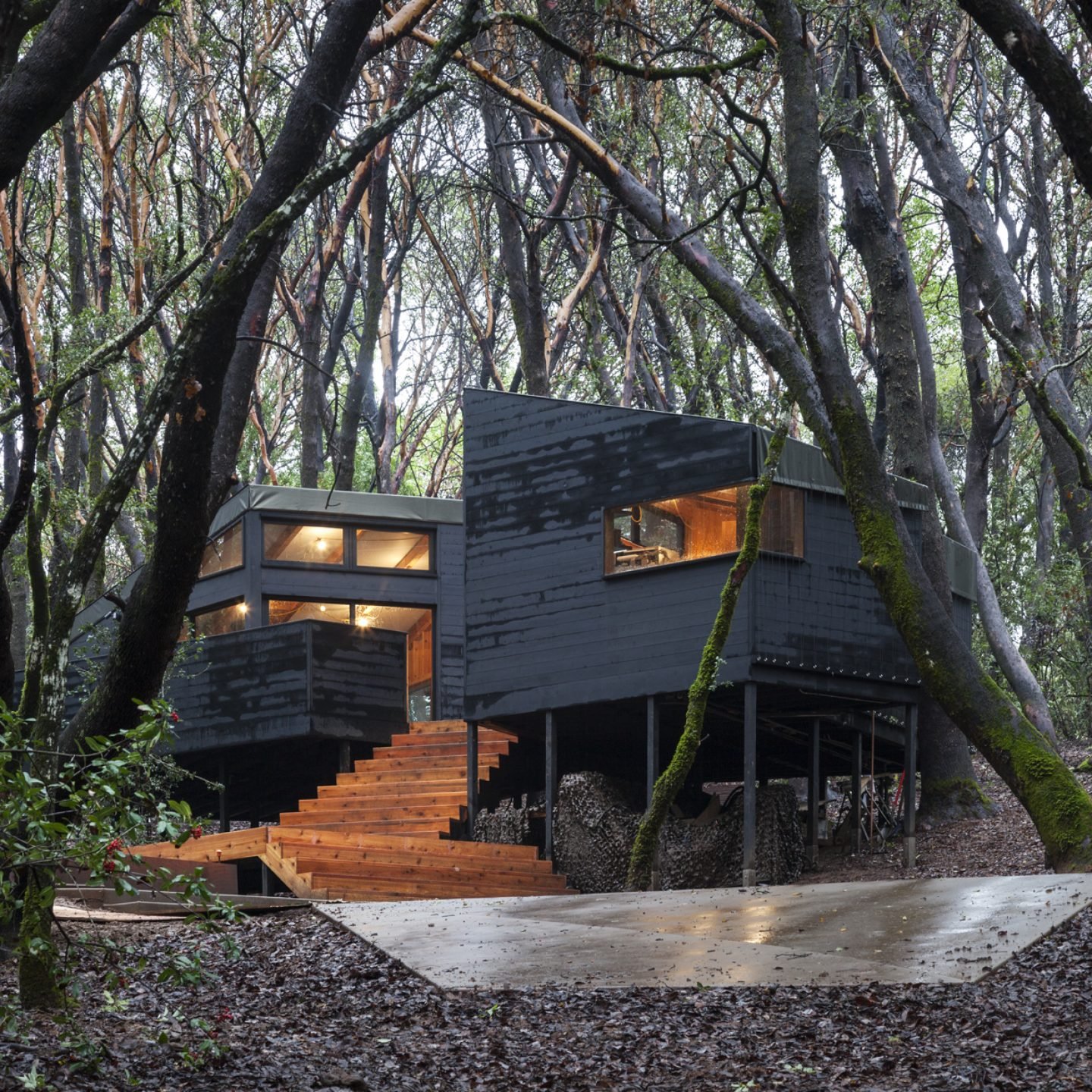This photograph captures a striking, modern house nestled amidst a dense forest, with a design that combines both architectural innovation and harmony with nature. The house is skillfully built into a hillside, elevated on stilts, giving it the appearance of a sophisticated treehouse. The exterior is clad in sleek black wood panels, enhancing its contemporary aesthetic, while the steps and some interior elements are in a warm cedar color, providing a pleasing contrast.

In the foreground, a small concrete driveway leads to a series of long, cedar-colored wooden steps, which appear wet as if it just rained. These steps ascend two levels between two separate, yet connected home-like structures. The main structure on the right, with its sharp angles and multitude of horizontal windows, exposes glimpses of the interior’s cathedral ceilings with white and wooden joists. The house's thoughtful, angular design and expansive windows allow it to blend seamlessly into its environment, while the thick tree cover provides seclusion and shade.

Overall, this modern architectural home creates an elegant balance between sleek, contemporary design and the tranquil, natural beauty of its forest surroundings.